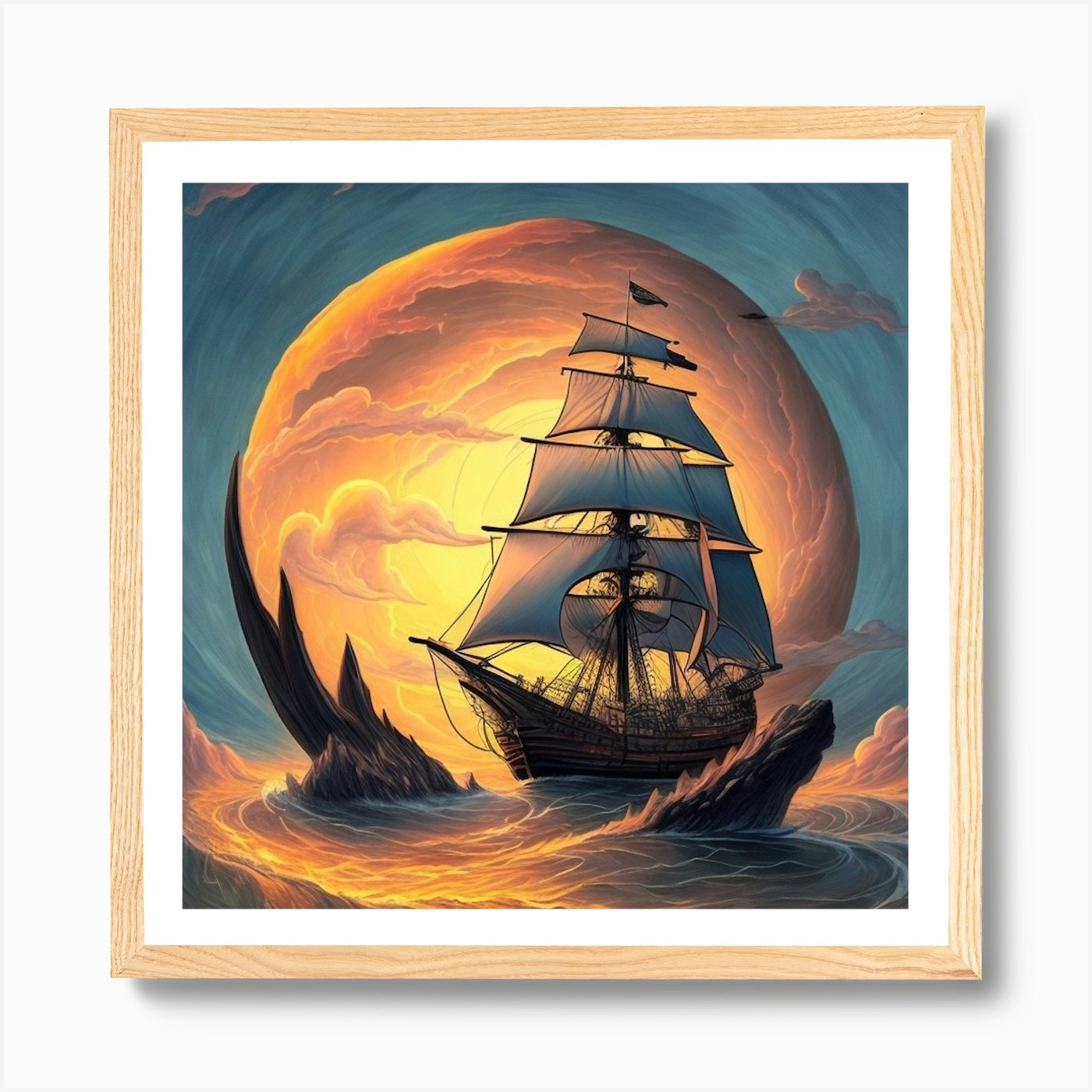This surrealistic and vividly detailed painting portrays a sailboat navigating through tumultuous, yellow-tinted waters under a giant, cloud-speckled white moon. The sailboat, crafted from wood, features a large, four-layered sail that shows signs of wear and tear, with oddly missing sections hinting at an AI-generated touch. The ship is detailed with symmetrical sails and mountain netting connecting the mast to its body, emphasizing its rugged and mystical nature. It sails toward the viewer, facing the treacherous passage framed by rocky, thorny, bark-like appendages jutting out from the churning sea, which almost appear to have teeth. The moon behind the boat, partially shrouded by clouds, exudes intense hues of yellow and orange, contrasting against the blue, vortex-like sky, adding to the painting's fantastical atmosphere. Framed elegantly with a wooden frame and a white mat, this artwork strikingly combines elements of danger and fantasy with its bold colors and intricate details.